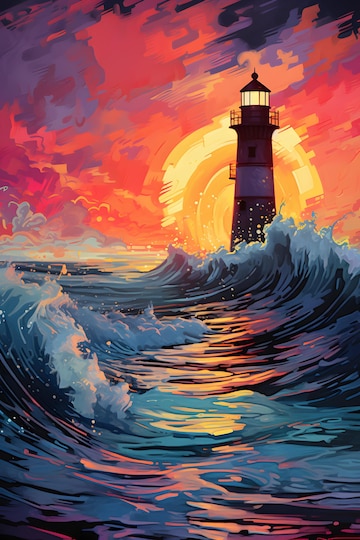The digital artwork vividly captures a dramatic lighthouse scene at sea during sunset. In the center-right, a dark red lighthouse with a prominent white stripe stands majestically, with its top section illuminated by a yellow light through its glass windows. The lighthouse is slightly shadowed due to the setting sun behind it, which radiates in concentric circles of orange and yellow, gradually transitioning into peach, pinks, and deep purples as it stretches across the sky to the darker blue corners. Below, the sun casts a brilliant reflection in streaks of yellow and pink across the water, adding a touch of realism. Surrounding the lighthouse, powerful waves with white caps crash against the shore from the right and appear to be coming inland from the left, creating dynamic U-shaped troughs. The image exudes a mesmerizing blend of vibrant and dark colors, portraying a serene yet powerful coastal scene enveloped in the vibrant hues of sunset.